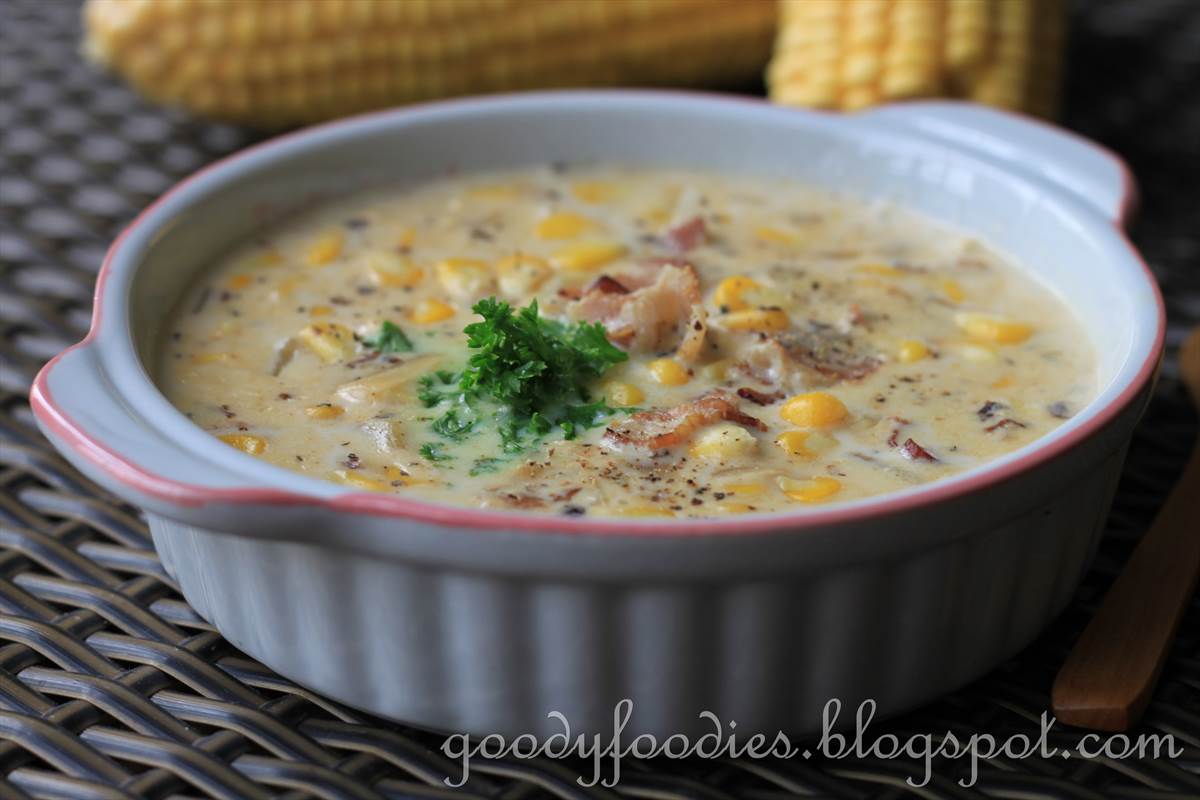The image is a rectangular photograph measuring about six inches wide and four inches tall, taken indoors. It is a close-up of a food dish, specifically a light yellow soup with visible ingredients including golden corn, possible chunks of meat like bacon or fish, small bits of green garnish likely parsley, and dark specks of seasoning, likely pepper. The soup is contained in an oval-shaped, fluted white casserole dish with a distinctive light pink-red stripe painted around the top rim and comes with two side handles. The dish sits on a black wicker-weave placemat. In the background, two peeled ears of corn on the cob are visible, blurred slightly, stretching from the left to the right of the top of the picture. At the bottom of the image, partly covering the wicker mat, lies the end of a wooden spoon. The lower right corner of the image features light gray cursive text that reads "goodyfoodies.blogspot.com," indicating the source of the picture.